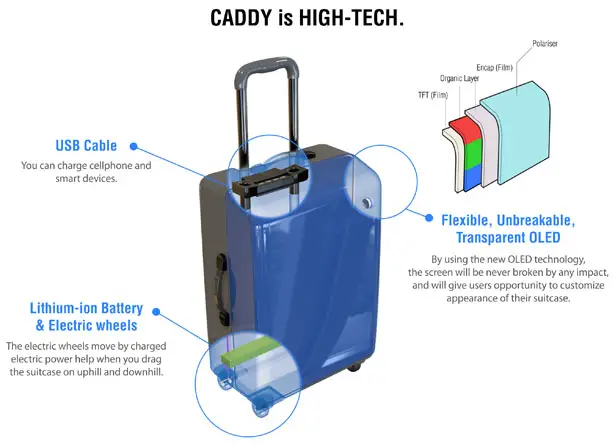This image is a detailed and high-tech illustration and graphic design in landscape orientation, showcasing a cutting-edge carry-on suitcase, referred to as "Caddy." At the center of the image is a black suitcase with an extended handle, depicted with a distinctive blue shadow. The suitcase is designed for modern travelers and features various innovative components. 

The top center text reads, "Caddy is high-tech," emphasizing the advanced nature of this suitcase. Several annotation blowout sections highlight its unique features: a USB cable plug-in for charging cell phones and smart devices, a lithium-ion battery powering electric wheels that assist in movement on inclines, and a revolutionary flexible, unbreakable, and transparent OLED screen. This OLED technology ensures that the screen will not break upon impact and gives users the option to customize the appearance of their suitcase.

The image also provides a detailed visual breakdown of the OLED screen’s construction, showing layers such as the polarizer, filter, organic layer, and film, each illustrated with descriptive text. The overall design blends sleek color illustrations with explanatory graphic design, presenting the Caddy as both a practical and technologically advanced travel solution.